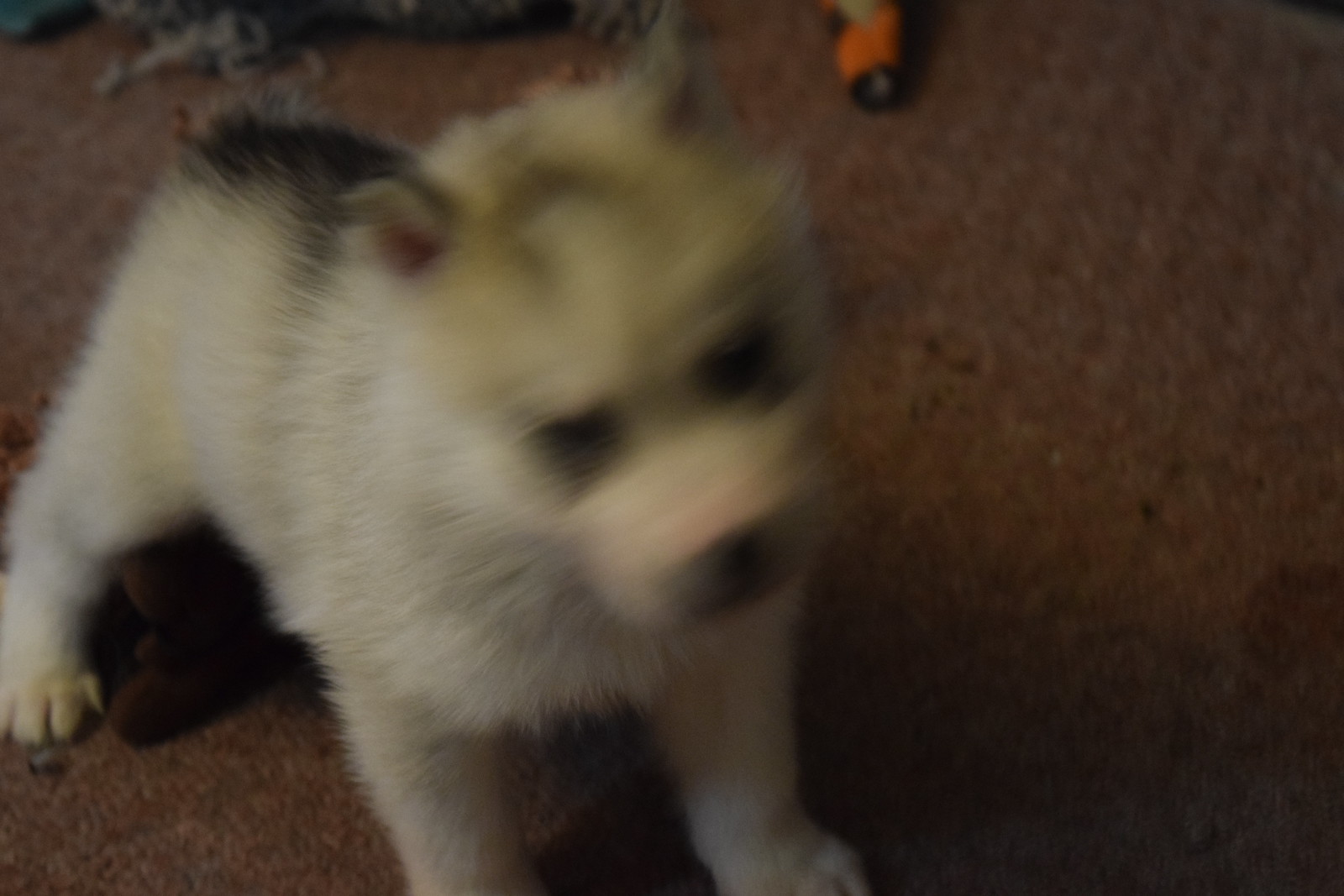In this rectangular, extremely blurred image taken in an indoor setting, we are looking down at a small cream-colored puppy with darkened ears. The puppy, positioned on a burgundy carpet, has pointy, upright ears and is facing forward. Its snout is black, and its dark eyes are surrounded by lighter areas. A distinct, upside-down U-shaped black marking adorns the puppy's forehead. In the upper right corner of the image, where the carpeting appears slightly brighter, a small, orange and black object extends from the top of the photo.